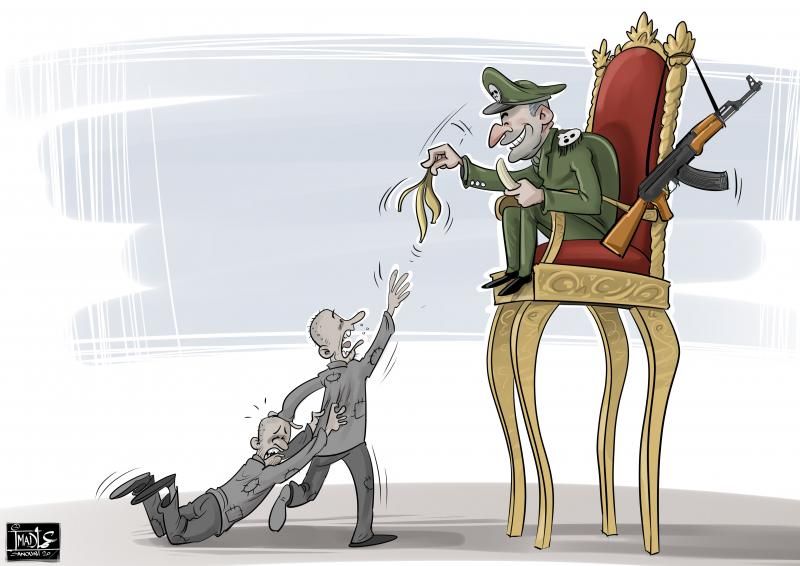This illustration depicts a scene with a striking contrast in power and desperation. On the right side, a man dressed in an olive green military uniform sits with authority on a grandiose throne-like chair that has long, ornate gold legs elevating him about six feet off the ground. The chair features a red cushion and backrest, giving it a regal appearance. A machine gun, possibly an AK-47, is hung menacingly from one of the chair's top pegs. The man, resembling a military dictator, holds a banana in his left hand and dangles a banana peel from his right, taunting two impoverished, raggedly dressed men below. These men, likely prisoners, have shaved heads and appear desperate and starving. One of the prisoners reaches out, mouth open and eyes pleading, for the banana peel, while the other, equally emaciated, clings onto his comrade's coat, partly lying on the gray floor. The entire scene stands against a simple blue background, emphasizing the stark contrast between the figures’ suffering and the dictator's opulence and indifference.